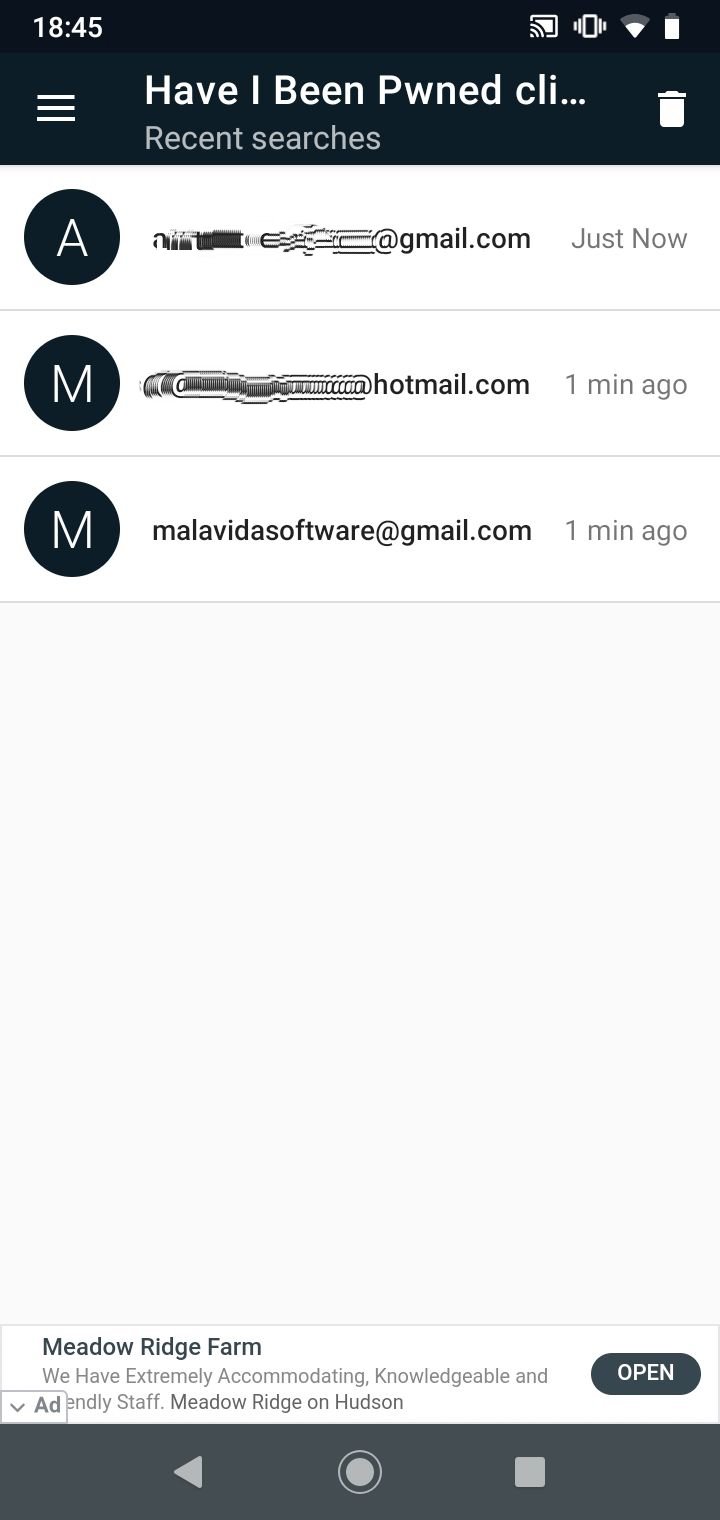The image captured is a vertically-oriented screenshot from a cell phone. At the very top, there is a prominent black horizontal banner that features various icons and indicators in white. On the upper left corner, the time is displayed as "1845" (6:45 PM). To the right, there is a sequence of icons: a cast icon, a cell phone vibrate icon, a Wi-Fi signal indicator, and a battery level icon. 

Directly beneath the time, on the left side, is a three-horizontal-bar menu icon, indicating a menu option. Centrally positioned, the text reads "I've been P W N E D," signaling a security or hacking-related application or notification. Below it, there is a section titled "recent searches," with a trash icon situated to the right.

The main content area displays three listings in white text. Each listing starts with a very dark gray circle containing a letter in white, aligned vertically from top to bottom. These letters are "A," "M," and "M" respectively. The listings are purportedly email addresses, with the first two distorted for privacy: the first ending with "@gmail.com" and the second with "@hotmail.com." The third, fully visible email address reads "malvitasoftware@gmail.com."